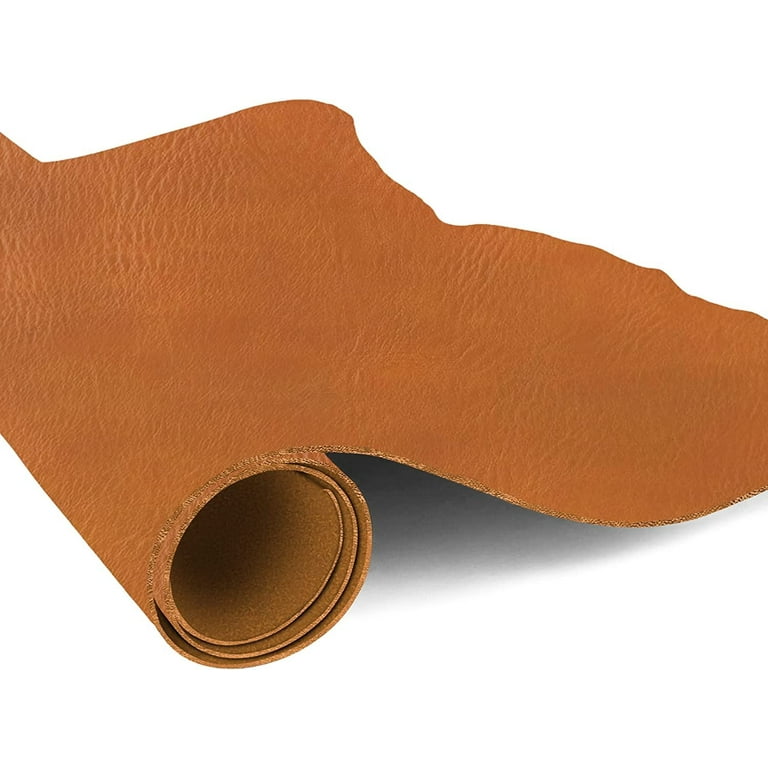The image depicts a digitized portrayal of a roll of leather, artfully highlighted against a stark, solid white background. The leather, painted a vivid orange-brown, is rolled 2 to 4 times before extending diagonally from the middle right and downward out of frame. The rolled leather exhibits a unique blend of smoothness and rough textures, indicated by various indentations and stretch marks. The edges where the leather unfurls are jagged and irregular, highlighting the natural grain, especially lighter where it has been cut. The roll casts a prominent shadow beneath it, adding depth to the predominantly bright scene. The object’s soft yet textured nature, with smoother bottom surfaces contrasted by the rougher inner folds, emphasizes its probable digital creation or significant digital alteration.